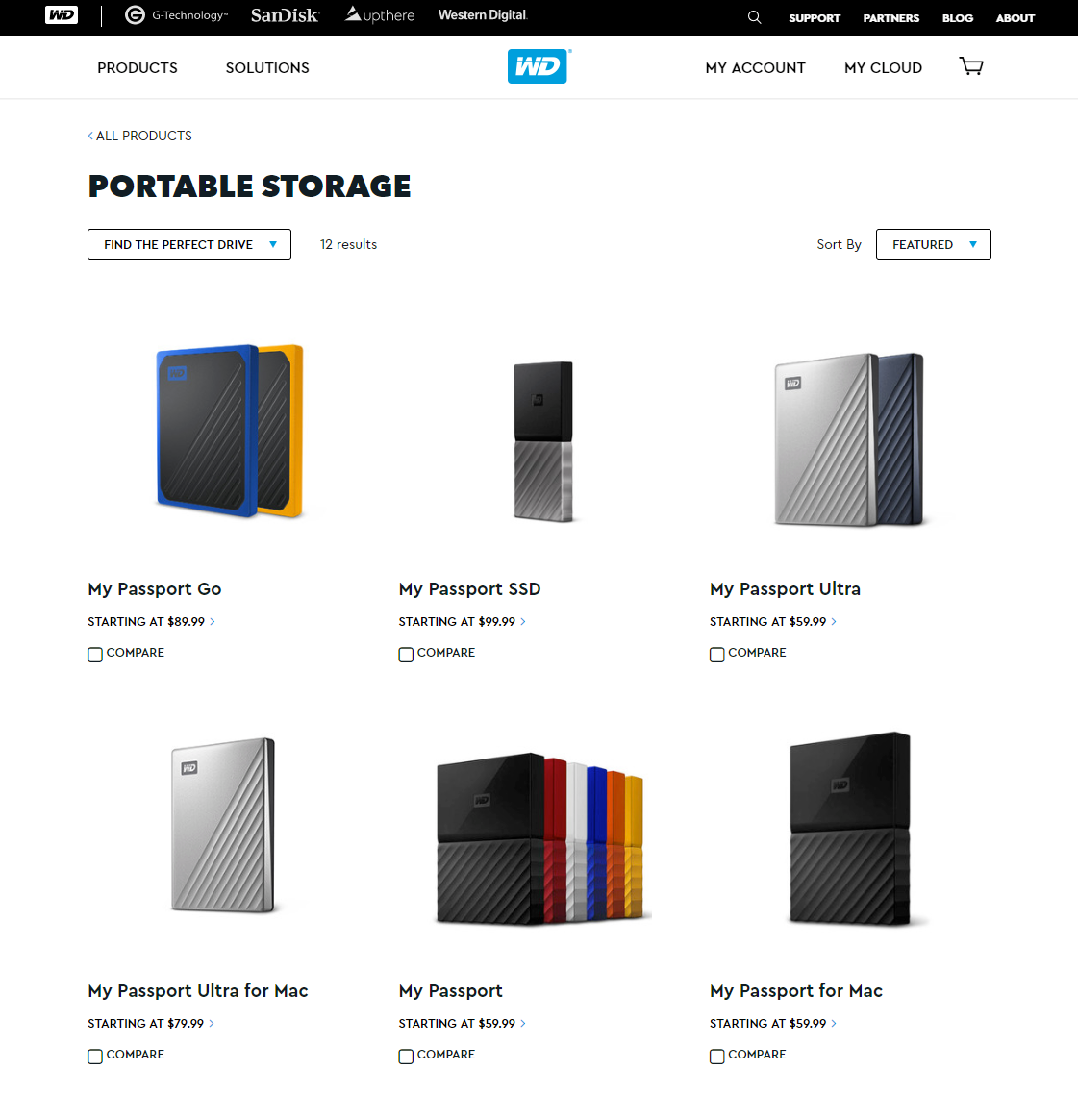This image is a detailed screenshot of the homepage of a website featuring Western Digital's product offerings. At the very top of the screen, the navigation bar displays several logos and links: a prominent "WD" logo inside a rectangle on the left, followed by the names "G-Technology," "SanDisk," and "Western Digital" in sequence. On the far right side of this top bar, there are buttons for Search, Support, Partners, Blog, and About.

Beneath this top bar, another navigation menu appears, listing options such as Products and Solutions on the left, with a central blue box containing the "WD" logo. On the right side of this menu, there are buttons labeled My Account, My Cloud, and a Shopping Cart icon for checkout.

The main content area below these navigation menus showcases various storage products with their descriptions and starting prices. The section titled "All Products, Portable Storage, Find the Perfect Drive" features several items:

1. **My Passport Go** (available in blue and yellow) starting at $89.99.
2. **My Passport SSD** (gray and black) starting at $99.99.
3. **My Passport Ultra** (gray and black) starting at $59.99.

On the bottom row:
1. **My Passport Ultra for Mac** (gray) starting at $39.99.
2. **My Passport** (available in black, red, white, blue, orange, and yellow) starting at $59.99.
3. **My Passport for Mac** (black) starting at $59.99.

The layout is designed to help users easily navigate and explore different storage solutions offered by Western Digital.